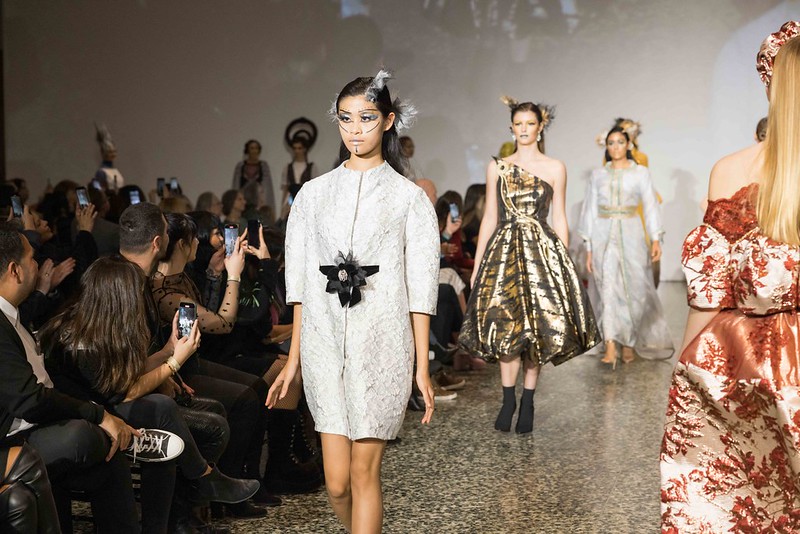This image captures an elegant and dynamic moment from a fashion show. Five models are positioned along the granite and marbled runway. The model at the front, of Asian descent, is wearing a short, white balloon-type jacket dress with sleeves reaching her elbows and a prominent black flower design at the waist. She also has decorative black and white ribbons or feathers in her hair, and delicate face paint with black lines adorning her cheeks and chin. Behind her, the second model dons a striking one-shoulder gold dress that balloons out at the bottom; she accessorizes with black shoes and gold and black ribbons in her hair. The third model is dressed in a flowing, sheer white and silver outfit, accentuated by gold ribbons in her hair. Moving further back, there's a glimpse of a fourth model in a golden leopard-patterned dress, while the model in the rear has a partially visible yellow dress. On the right side of the runway, another model is making her exit in a cream dress with red and orange floral patterns, complemented by a top ruffle.

To the left of the runway, rows of spectators are visible, impeccably dressed in black attire and eagerly capturing the show on their cell phones. The audience is seated in folding chairs, fully engaged in the spectacle before them. At the far end of the runway, a few models are seen waiting their turn, poised against a light tan background, adding to the anticipation and rhythm of the event.